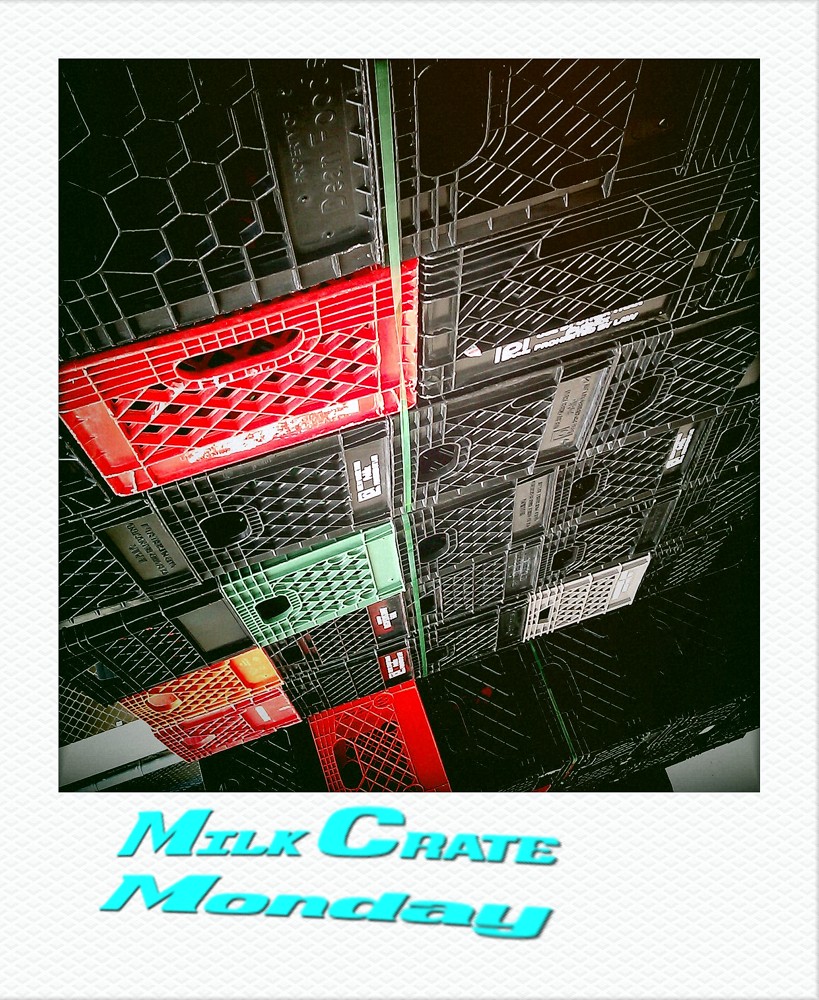The image features a striking array of at least 25 stacked plastic milk crates, displayed against a white backdrop. The crates, predominantly black with notable red and green variations, form an impressive wall-like structure. Each crate is adorned with a white logo and writing, indicating their dairy origins. To add to the visual intrigue, the crates are oriented in various directions, creating a dynamic and somewhat chaotic arrangement.

Beneath this central image, bold turquoise text spells out "Milk Crate Monday," slightly skewed to the left. This text along with the entire image is presented with a tilted theme, giving the photo a playful and whimsical feel. The overall aesthetic is reminiscent of a Polaroid or postcard, with a faint honeycomb pattern subtly visible in the white background.

The dark blue lettering, offset asymmetrically beneath the crates, emphasizes both the text and the colorful, jumbled assortment of milk crates, making the image a visually engaging composition.